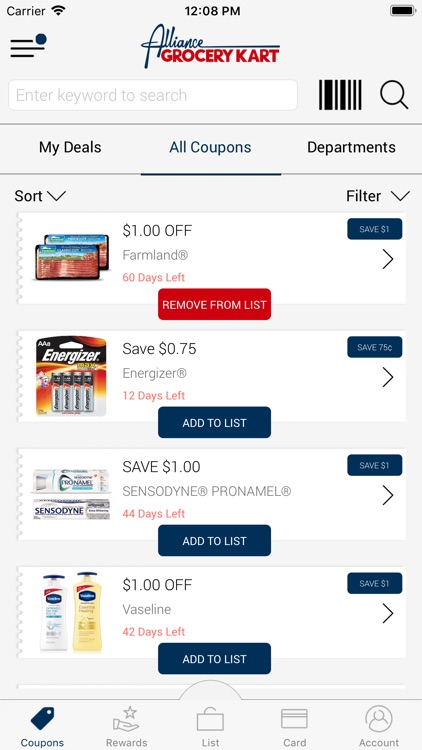Screenshot of the Alliance Grocery Cart Mobile App:

The screenshot depicts the user interface of the Alliance Grocery Cart mobile app, set against a light gray background. Centrally located is the company logo, with the word "Alliance" elegantly written in cursive blue lettering. Directly beneath the logo, "grocery cart" is printed in bold red letters, with a distinctive 'K' replacing the 'C' in "cart."

Below the logo is a functional search bar labeled "Enter keyword to search," accompanied by small icons of a barcode and a magnifying glass to assist with the search functionality. 

The navigation section follows, featuring prominent links for "My Deals," "All Coupons," and "Departments." In this particular screenshot, the user has selected "All Coupons." 

In the "All Coupons" section, there are two dropdown menus for sorting and filtering options situated to the left and the right, respectively. Below these options are visual representations of available coupons. The first coupon displayed is for Farmland bacon, offering $1 off and indicating it has been added to the list with an option to remove it. Other coupons visible include $0.75 off Energizer batteries, $1 off Sensodyne Pronamel toothpaste, and $1 off Vaseline lotion. Each coupon details the remaining days available for the discount and provides options to add or remove the coupons from the user's list. 

At the very bottom of the interface, there are additional navigation links for "Coupons," "Rewards," "List," "Card," and "Account," each labeled in clear blue lettering.